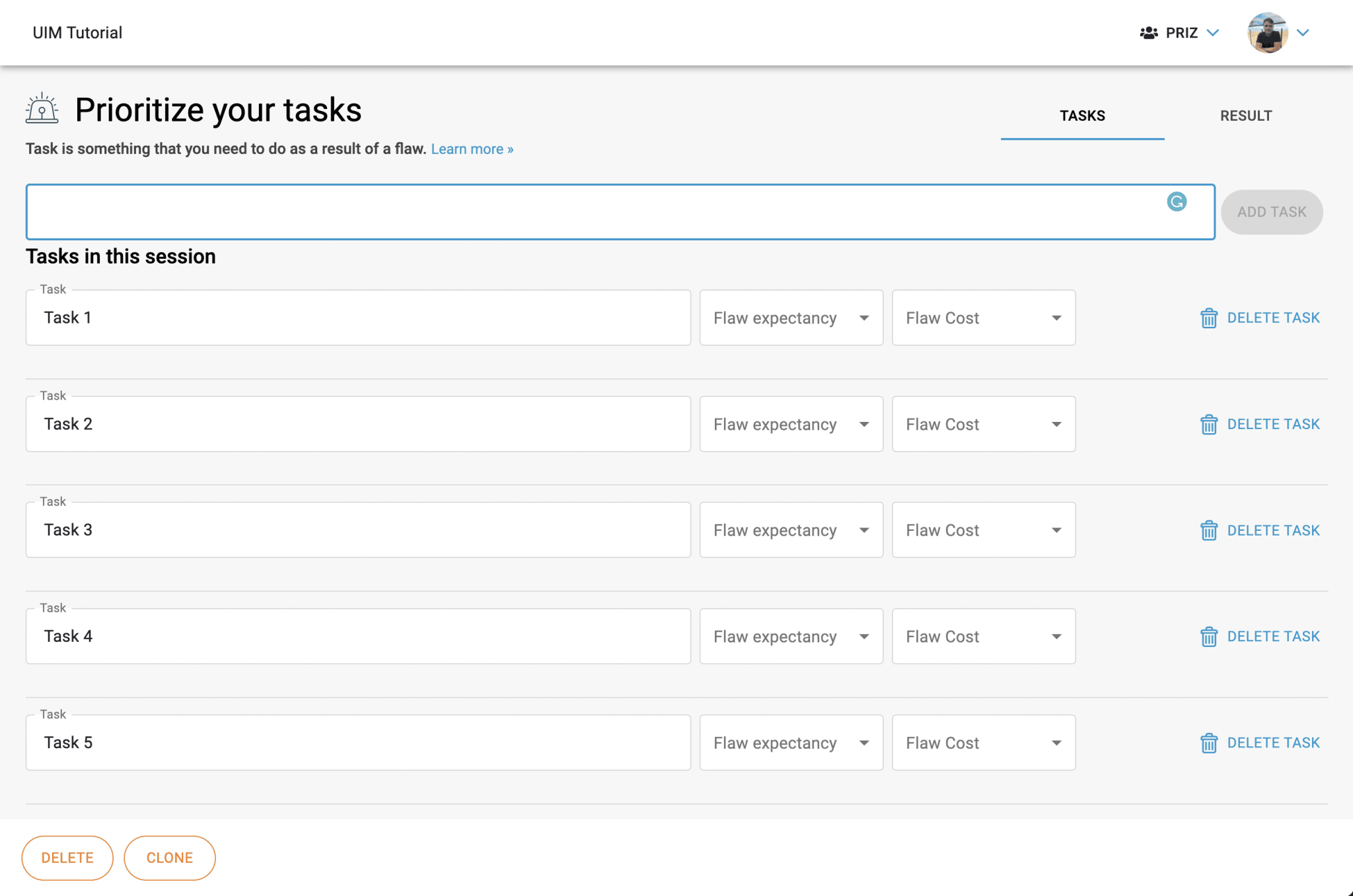The screenshot depicts an app interface designed for task management. The overall layout is wide and not very tall, with no visible device UI, suggesting a web application or software platform. 

### Header Section:
- **Background**: White rectangle spanning the top as the header.
- **Left Side**: 
  - Black text that reads "UIM tutorial".
- **Right Side**: 
  - A black icon depicting three people.
  - Text next to the icon reads "PRIZ".
  - A blue downward arrow follows the text.
  - Next, a small circle contains an avatar—likely a person's upper half against a background.
  - Another blue downward arrow is beside the avatar.

### Main Body:
The content area below the header has a light gray background and is organized as follows:

- **Top Left Section**:
  - Large heading text reads "Prioritize Your Tasks" in black.
  - An icon to the left of this text resembles either a light bulb or a half-circle with lines.
  - Below this heading is a subheading in smaller text that reads "Task is something that you need to do as a result of a flaw."
  - The phrase "Learn more" is in blue, indicating a clickable link.

- **Top Right Section**:
  - Text that reads "Tasks" in black, with "Result" in gray next to it. 
  - The "Tasks" option appears selected, indicated by a blue underline.

- **Task Input Area**:
  - Below the top sections is a white, outlined rectangle with a blue border across the screen.
  - On the right side of this rectangle is an "Add Task" button, currently inactive as no text has been entered.

- **Task Rows**:
  - There are five rows numbered from Task 1 to Task 5, which include:
    - A white rectangle containing the task name.
    - To the right, dropdown menus labeled "Flow Expectancy" and "Flow Cost."
    - A blue trash can icon labeled "Delete Task" for removing tasks.

### Bottom Section:
- **Left Corner**:
  - Two orange outline buttons with white backgrounds:
    - "Delete" on the left.
    - "Clone" on the right.

Overall, the screenshot showcases a clean, function-oriented interface tailored for task organization and management with intuitive navigation and actionable options.